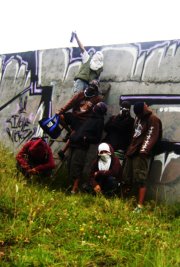The photograph depicts six individuals, predominantly men, gathered in front of a stone wall that is covered with a mix of blue, white, gray, and black graffiti. The wall stands adjacent to a field with unkempt green grass. The group, characterized by their varying attire of hoodies with large hoods, long pants, jeans, cargo shorts, and face-covering masks in black and white, gives an impression of unity amidst anonymity. Some members are actively tagging the wall with spray paint. One individual is crouched down, another is hiding his face, while one observer looks directly at the camera. Notably, one person in brown attire is seen helping another in white and dark green reach or climb the wall, presumably to access a higher section for graffiti. An additional figure, distinct in red clothing, sits towards the left-hand side of the image.